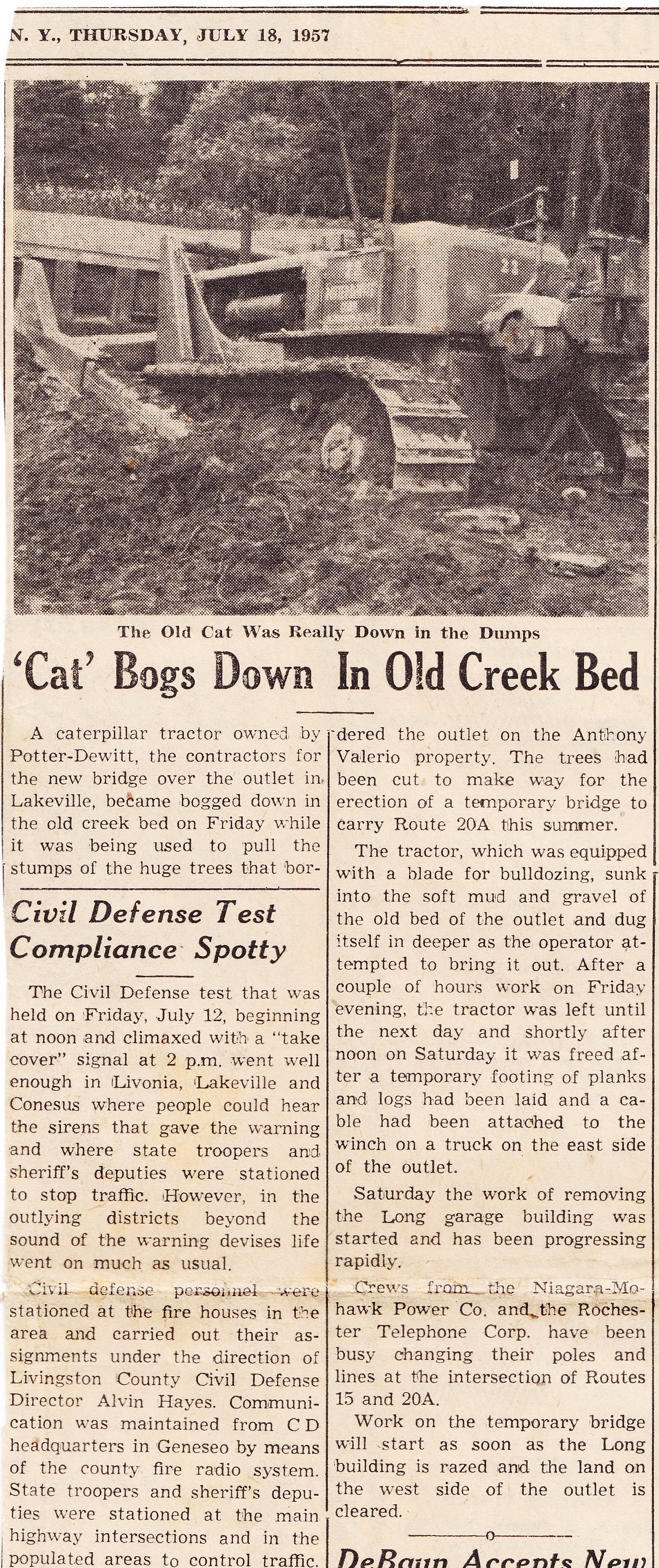This is a detailed rectangular vertical image of a vintage newspaper clipping dated Thursday, July 18, 1957. Dominating the upper part of the clipping is a black and white photograph depicting a large piece of machinery, likely a Caterpillar tractor, stuck in a muddy creek bed. The headline beneath the photo reads, "Cat Bogs Down in Old Creek Bed," with "Cat" in quotation marks to signify it's a Caterpillar brand tractor. This incident involved a Caterpillar tractor owned by Potter DeWitt, contractors for the new bridge over the outlet in Lakeville. The tractor became bogged down in the creek bed on a Friday while pulling stumps of huge trees on the Anthony Vallejo property. These trees were cleared to erect a temporary bridge for Route 20A during the summer. The newspaper’s color palette includes shades of white, tan, black, and various grays, consistent with the print styles of the 1950s. Below the primary article, minimal text is visible, but it mentions another headline, "Civil Defense Test Compliance Spotty," reflecting on a civil defense test held on July 12, which went well in specific areas but was less effective in outlying districts. The newspaper article and its accompanying details highlight the events in a snapshot of historical reportage.